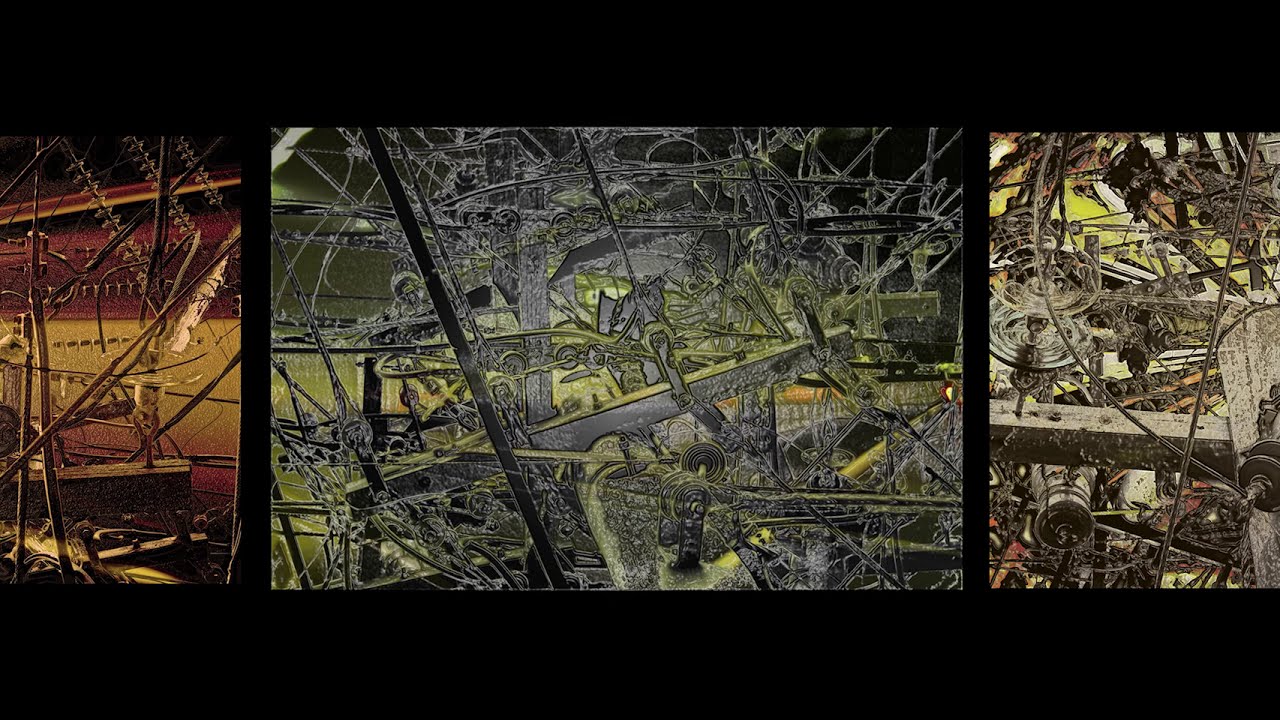The image features three distinct sections, each composed of a chaotic array of objects that evoke the feeling of a scrapyard. The left section presents a predominantly dark-themed assortment with a color palette of brown and dark golds, against a backdrop hinting at red and yellow hues. This area is filled with what appears to be tangled wiring and metal rods, lending it a slightly industrial yet chaotic aesthetic.

The central section stands out with its full rectangle composition, showcasing a clutter of gears, hammers, motors, pistons, and even a pulley, all in a color palette dominated by green and silver, with a hint of black. This section resembles an intricate, disordered erector set, reminiscent of dismantled scaffolding scattered about.

On the right, the section is characterized by a brown and yellow theme, with maroon and orange undertones. It contains circular metal objects that seem to be part of a varied assortment of rectangles, suggesting old screws or turbines. The entire image, though abstract with strong lines going in every direction, depicts a technological and mechanical scene, blending elements that appear to be either from a construction site or a deconstructed piece of machinery.